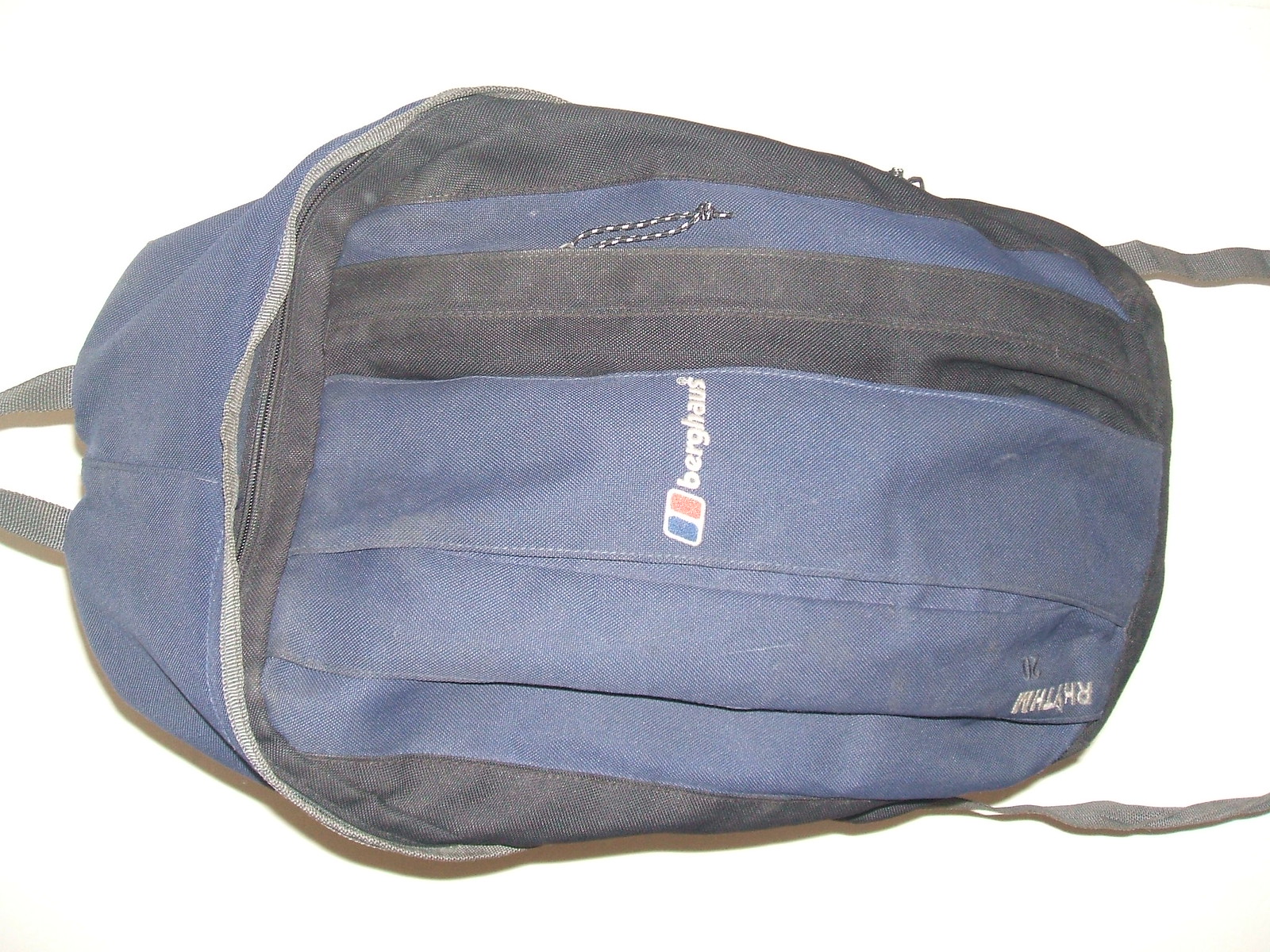This image depicts a blue backpack made of canvas-like material, lying horizontally against a white background. The top of the backpack is positioned on the left, with its black shoulder straps extending towards the left side, close to the center of the image. The main compartment of the backpack features a gray flap covering a black zipper that encircles the bag. 

The front of the backpack displays the brand name "Berghaus" in white letters, flanked by a logo with two rounded rectangles—one red and the other bright blue, distinct from the darker navy blue color of the backpack itself. Lower down on the bag, partially obscured by folds, is another word printed in black that says "Rhythm," though it appears upside down. 

Additional details include black and silver trim around the zipper area, white and black ties on the zippers for easy opening and closing, and two black straps extending from the right side of the backpack. The bag shows signs of wear and dirt, adding to its rugged appearance.